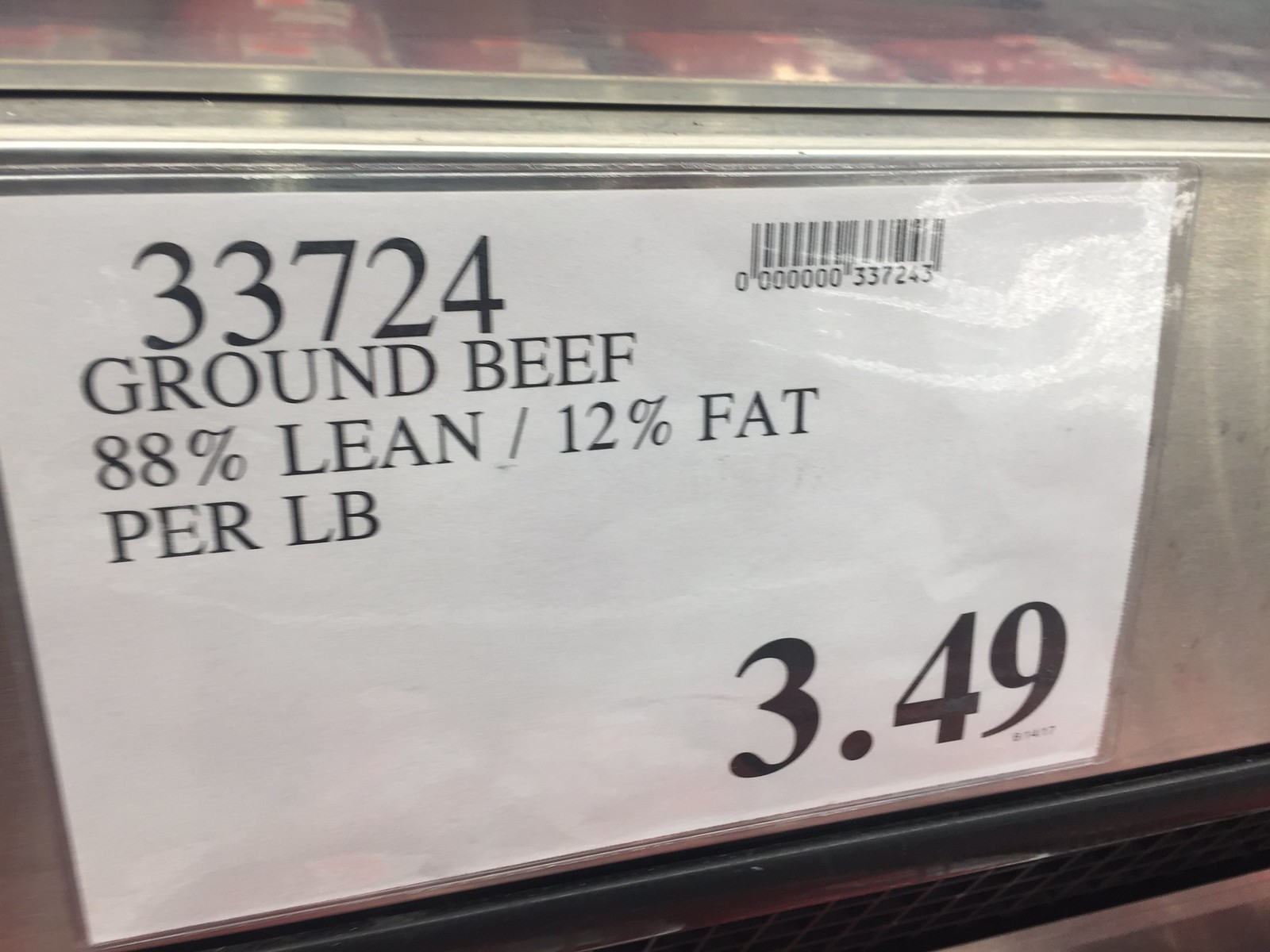This is a close-up image of a price tag on a metal shelf in a grocery store, specifically within the meat section. In the background, packages of red meat can be seen in clear packaging. The shelf itself is silver metal with a black border, and a portion of the floor is visible at the bottom of the frame. The white price tag is inserted into a plastic cover attached to the metal shelf, allowing for easy updates. The tag features black capital letters and includes a barcode on the right side. The text reads "33724 Ground Beef 88% Lean 12% Fat Per Pound." The most prominent detail is the price displayed in large black numbers: $3.49.